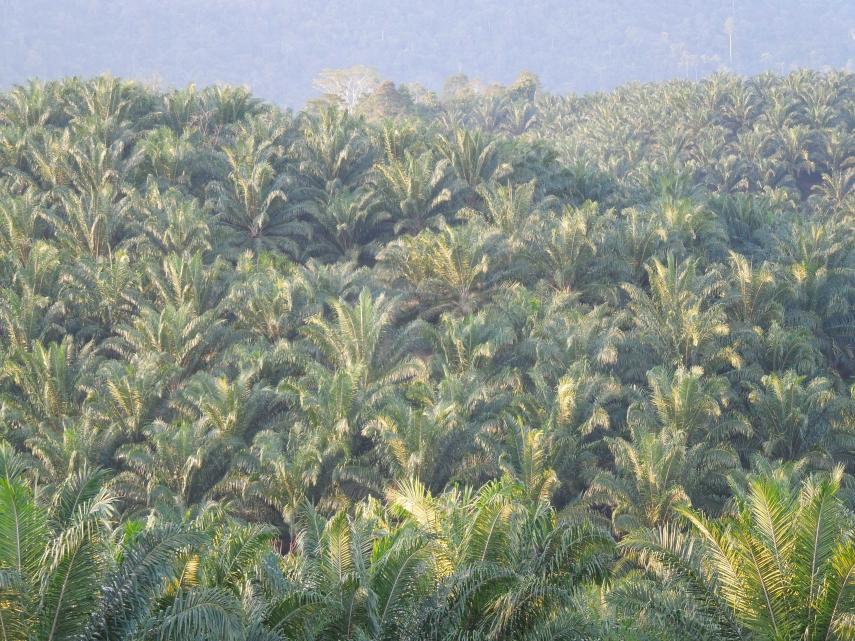This image captures a vast, tropical forest canopy spanning from the bottom to almost the top edge of the frame, with the leaves densely packed and predominantly green. The canopy appears to consist of palm or similar tropical foliage, forming an expansive, lush green cover that's consistent throughout its span. A notable gray mist or haze overlays the scene, casting a soft, smoky appearance over the treetops. Light from the sun filters through the dense foliage, creating subtle shadows and highlights, primarily at the topmost parts. In the distant horizon, there's a visible dip in the landscape, leading to a secondary, less distinct tree line, likely blurred and muted by the same gray haze that defines the upper section of the image. Among the primarily uniform tree line, there are a few distinguishable evergreens, particularly towards the right, where one stands more prominently against the dim background.